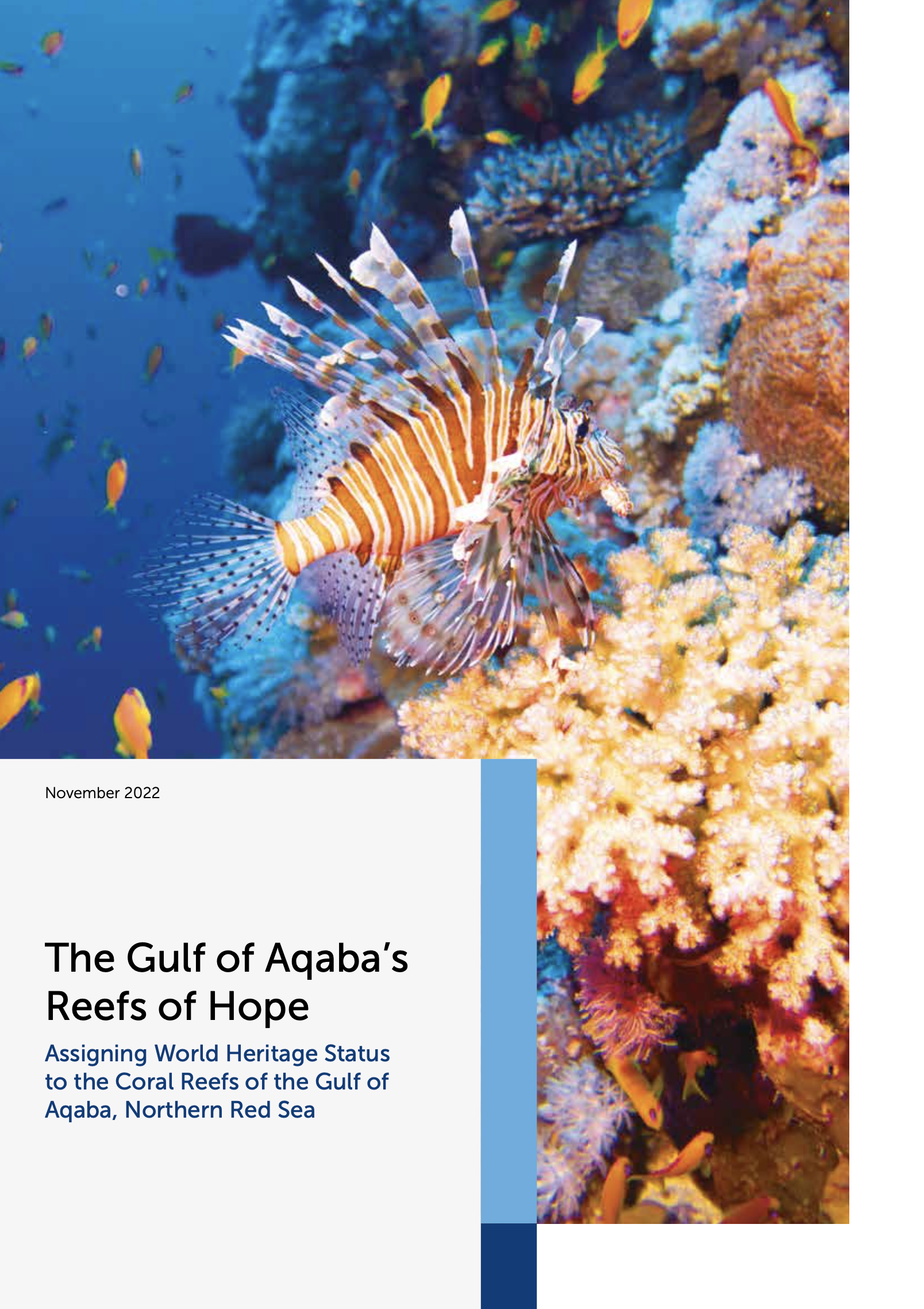This underwater photograph captures a vibrant scene from the Gulf of Aqaba's Reefs of Hope, part of the coral reefs of the Northern Red Sea. Central to the image is a striking fish, possibly a lionfish, characterized by its orange, yellow, and white stripes along its body and elongated, fin-like appendages that fan out dramatically. Surrounding the fish is a wall of diverse coral reefs, displaying an array of colors including prominent yellow and orange corals near the fish. Also visible in the photo are small yellow and orange fish swimming around, adding to the lively underwater tableau. The background features the deep blue underwater expanse with scattered rocks and additional corals. In the lower left corner, a light grey text box contains the caption: "The Gulf of Aqaba's Reefs of Hope," followed by the subtitle in dark blue font, "Assigning World Heritage Status to the Coral Reefs of the Gulf of Aqaba, Northern Red Sea." The photo is also timestamped "November 2022."